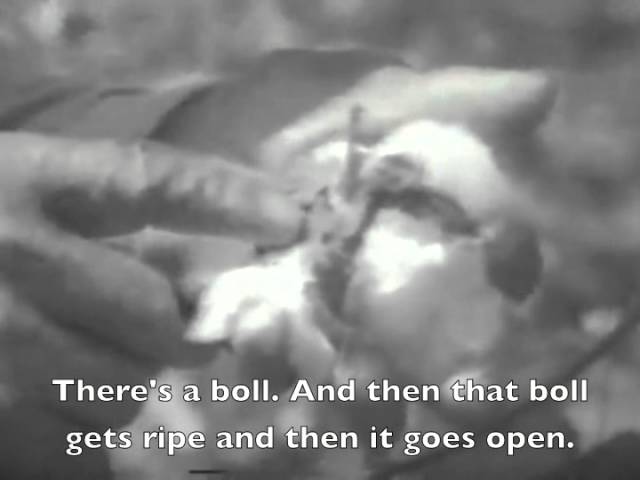This is a black-and-white photograph, approximately 5 inches wide and 3 to 4 inches tall, featuring a somewhat blurry image of a cotton bulb at its center. The cotton, identifiable by its rounded white poof and attached seed pods, is held by two hands entering from the left side of the image. The left hand cups the cotton while the right hand points to a specific part of it, specifically focusing on the seed. The image serves an explanatory purpose, further emphasized by the text at the bottom. In two rows of white text outlined in black, it reads: "There's a bowl, spelled B-O-L-L, and then that bowl gets ripe and then it goes open."